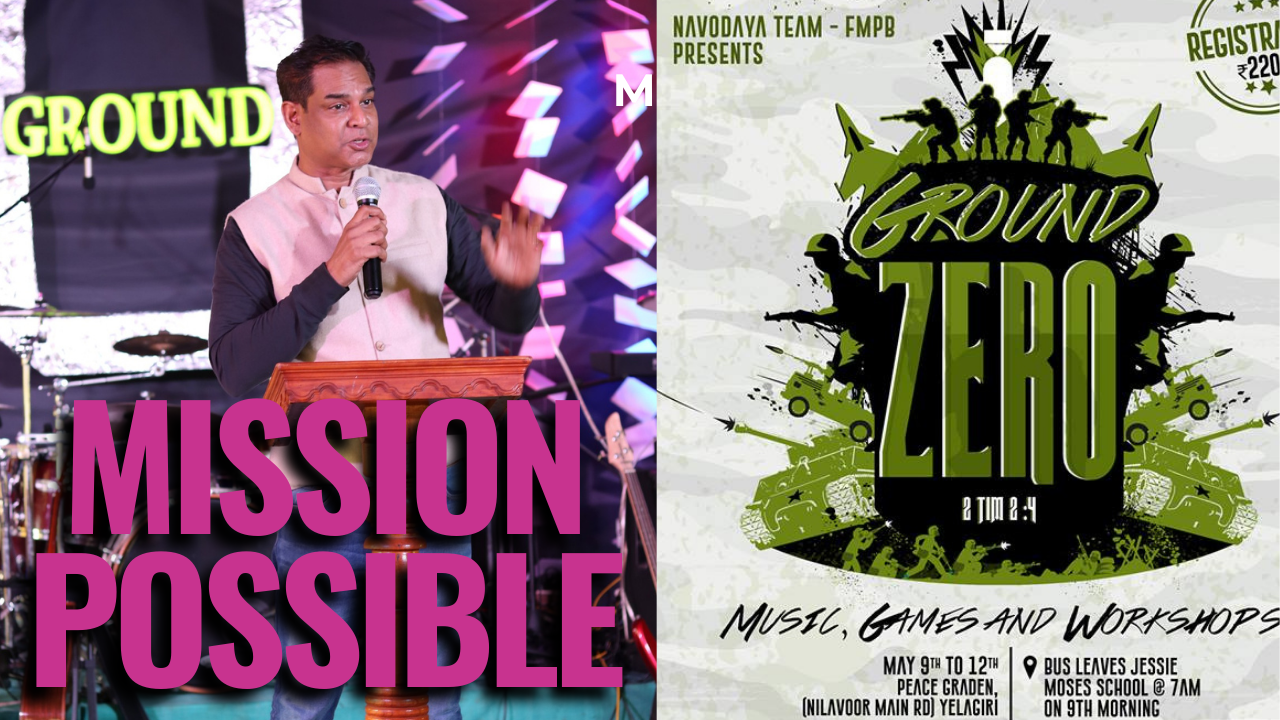This image appears to be a collage promoting a religious festival, featuring two distinct photos on the left and right sides. The left side of the collage shows a man standing at a podium with a microphone in his hand, wearing a white vest over a long blue t-shirt. He appears to be delivering a presentation or sermon, with vibrant and wild colors in the background, including a possible drum set behind him. Yellow lettering spells out the word "ground" next to his head, while large purple font in front of him reads "Mission Possible."

On the right side of the collage, there is an advertisement for the festival titled "Ground Zero." This ad promotes music, games, and workshops, and specifies the event dates as May 9th to 12th at Peace Garden. Additional details include that a bus will leave Jesse Moses School at 7 a.m. on the morning of May 9th and mentions that registrations are now open. The primary colors of the festival ad are green and black.